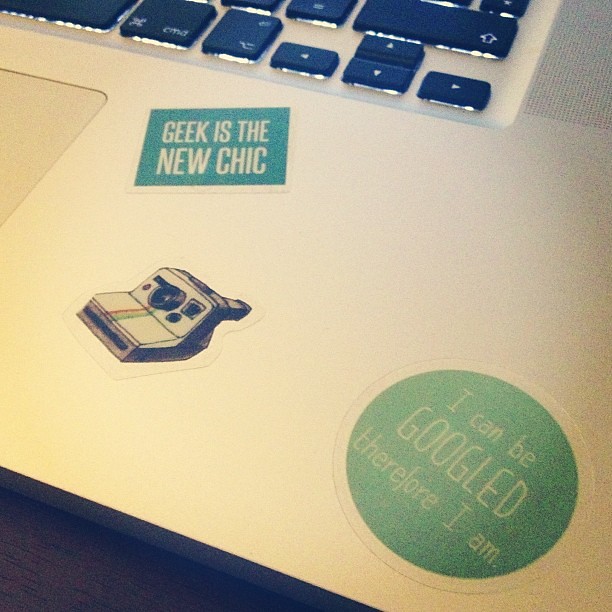The image is a large, somewhat blurry square close-up of a laptop's lower section. At the upper part of the image, you can see the black keys of the illuminated keyboard, specifically the arrow keys and the enter button. The right edge reveals a small section of the mousepad. The silver base of the laptop displays three distinct stickers: the first one, positioned at the top, reads "Geek is the New Chic" in all caps with white letters against a teal green background and a white border; the second sticker, in the middle, features a Polaroid camera with rainbow colors streaming down; and the third one, located in the lower right-hand corner, is a circular sticker with a white border that says "I Can Be Googled, Therefore I Am" in white text on a green background. Additionally, a small portion of a brown desk is visible at the bottom left corner of the image.